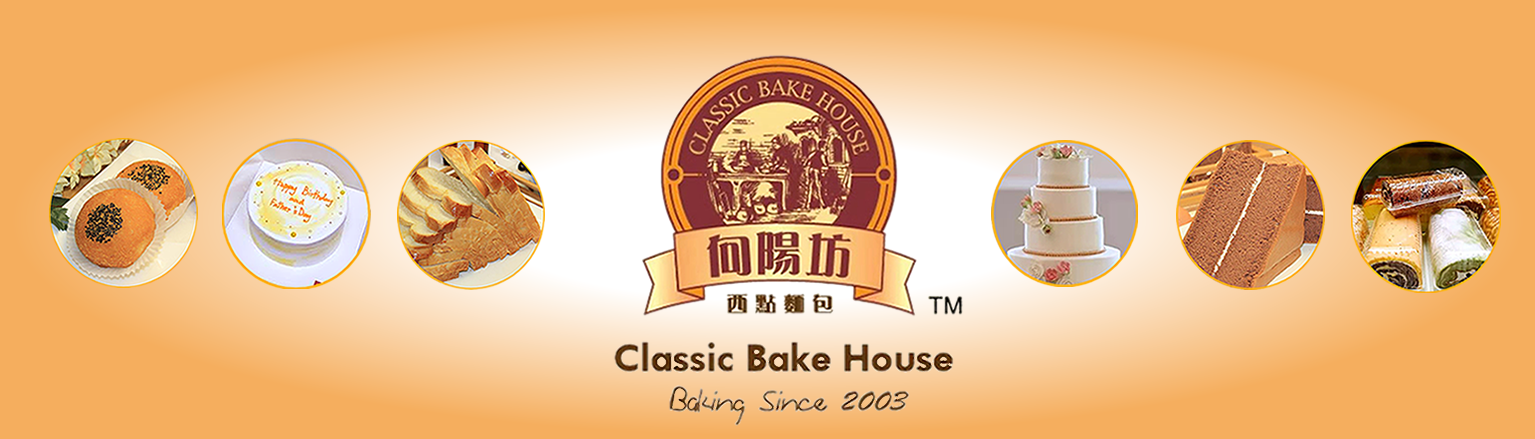The image is a wide, horizontal rectangular banner for the company Classic Bakehouse, intended for a website. The background features an orange gradient that transitions from a white glow in the center to a deeper orange at the edges. Central to the banner is a circular logo with "Classic Bakehouse" inscribed within. The logo consists of a yellowish center bordered by a dark brown rim and a thinner golden rim. Below the logo is a ribbon containing Japanese characters, and the text "Classic Bakehouse - Baking Since 2003" appears beneath that.

Flanking the central logo are six circular photographs of various baked goods, three on each side. From left to right: two light brown buns topped with black seeds, a white birthday cake with orange writing, and a loaf of white bread sliced. On the right, the images depict a four-tiered white wedding cake, a slice of light brown chocolate cake with a white frosting layer, and three sweet rolls in clear plastic containers. This detailed banner harmoniously combines visual elements to showcase the brand and its confectionery offerings.